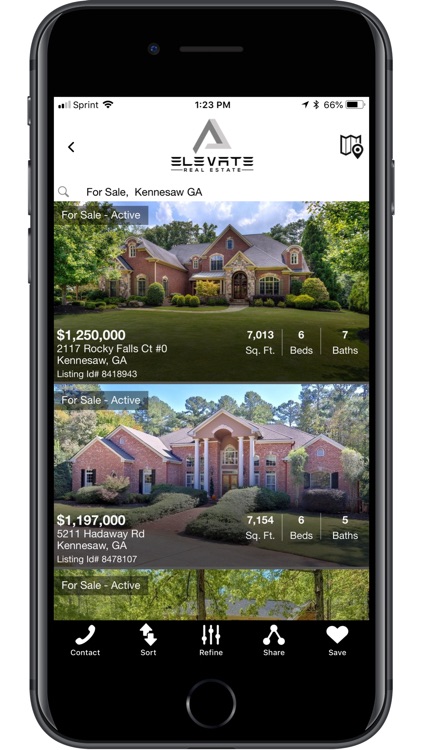The image is a detailed screenshot of a smartphone displaying a real estate app interface. At the upper edge of the screen, the status bar shows the network carrier "Sprint" on the left, the time "1:23 PM" in the center, and the battery level at "66%" on the right. Below this, the app's header reads "Elevate Real Estate," indicating the user is searching for properties in Kennesaw, Georgia.

The main body of the screenshot showcases two high-end property listings. The first property is a magnificent brick house priced at $1,250,000. It features 7,013 square feet of living space, 6 bedrooms, and 7 bathrooms, located on Rocky Falls Street in Kennesaw, Georgia. The house appears to have two to three levels, enhancing its grandeur.

Beneath it is another luxurious listing priced at $1,197,000. This house offers 7,154 square feet of living space, with 6 bedrooms and 5 bathrooms, also located in Kennesaw, Georgia. The image displays part of a third listing, hinting at additional properties available in the search results but not fully visible in this screenshot.